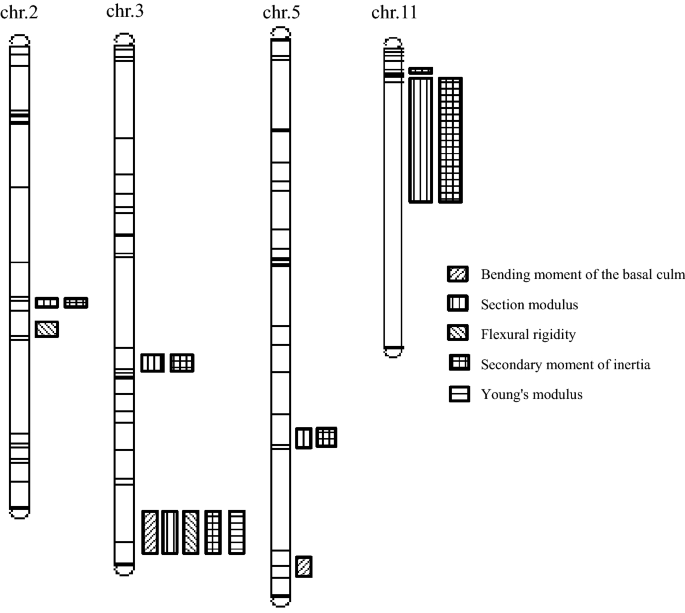The image is a black-and-white textbook diagram depicting a detailed scientific explanation, possibly related to physics or materials science. The central elements are four vertically oriented bar charts, each labeled with "CHR" and numbered 2, 3, 5, and 11. These bars vary in length and have horizontal lines running across them, which correlate with specific properties listed in the legend on the right side of the image. The legend details the various sections and lines, identifying them as the bending moment of the Basal comb, section modulus, flexural rigidity, secondary moment of inertia, and Young's modulus. The combination of the numbered bars and the descriptive legend suggests that this diagram is used to illustrate different mechanical properties or behaviors of materials, with each bar representing specific measurements or characteristics outlined in the legend.